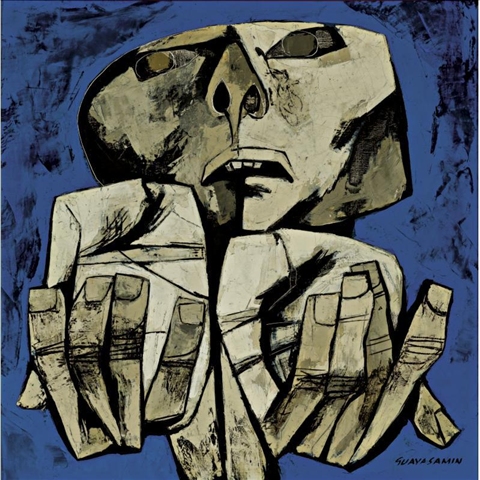This artwork, created by the artist Guava Salmon, features a style reminiscent of Picasso with a hint of cubism. The composition is square and includes a signature in black on the bottom right. The piece depicts an abstract human form, focusing on a large head and two prominent hands with palms exposed and fingers curling upwards. The head, placed at the center top, has an open mouth in a halfway frown revealing four protruding teeth, and wide-open eyes with smudged brown pupils and white circles indicating the eye position. The face is elongated, resembling an upside-down triangle, and conveys an E.T.-like appearance with large eyes, a defined nose with two nostrils, and a bold, outlined mouth.

The figure, rendered primarily in varying shades of grey, black, brown, and beige, appears almost rock-like with a carved texture. The hands, also in neutral tones, feature long, square fingers with flat nails. The body below the head is partially visible, with legs somewhat obscured, maintaining the focus on the upper section.

The vibrant blue background, enhanced with black smudges around the edges, adds depth and texture to the scene, contrasting the neutral hues of the figure, and framing the stark, bold lines that define the abstraction.